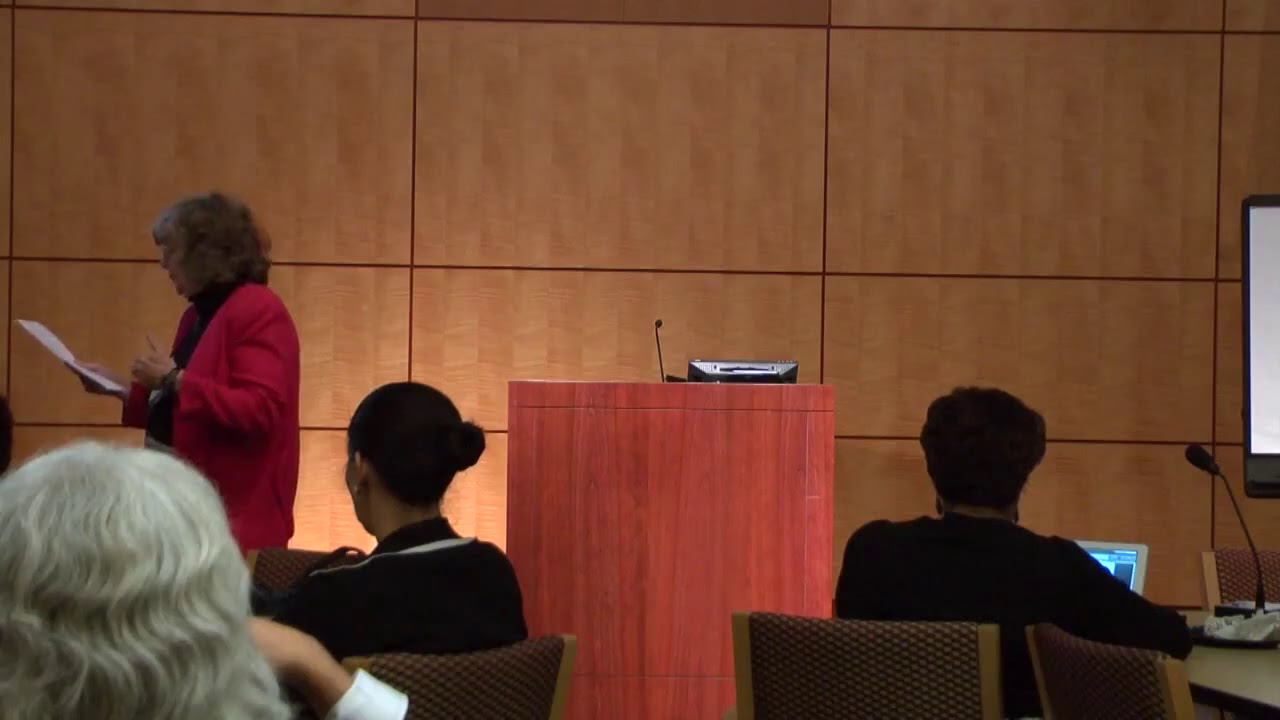In the image, the focal point is a cherry-red wooden podium positioned centrally, equipped with a small microphone at its center and an ambiguous electronic device with buttons and a handle on its top right, resembling a horizontal boombox. The backdrop features light brown wooden or faux wooden tiles. To the left of the podium, a woman with long, shoulder-length curly hair, graying brunette in color, is turned side profile to the camera. She is wearing a red blazer over a white turtleneck shirt and is examining a piece of paper or pamphlet in her hands. In the foreground, three audience members face the woman. On the bottom left, a woman with long gray hair sits facing away from the camera. In the center left, another woman with jet black hair styled in a bun, dressed in a black jacket, is visible. To the center right, a third woman, with short black hair and clad in a black top, is working on a laptop, which is positioned next to a microphone seen at the bottom right of the image. The edge of a digital slideshow presentation screen is slightly visible at the middle right.